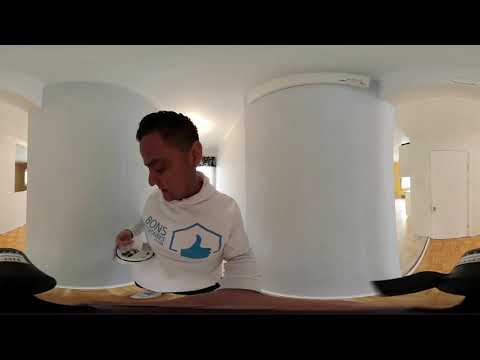The image showcases a 360-degree VR view of a room with a fair-skinned man holding a flat, circular object, likely a smoke detector, close to his chest. He is dressed in an all-white hoodie featuring a blue thumbs-up icon inside a basic house-shaped outline. Below this logo, the capitalized letters "B.O.N.S" are prominently displayed. The setting includes white walls, doors, and possibly some distortion leading to the appearance of two large circular columns. Behind him, there are three hallways; the left hallway shows a window partially, the central hallway has sunlight streaming in through another window, and the right hallway leads to a closed door. The scene is framed with a wooden floor and some black objects on both ends of the image.